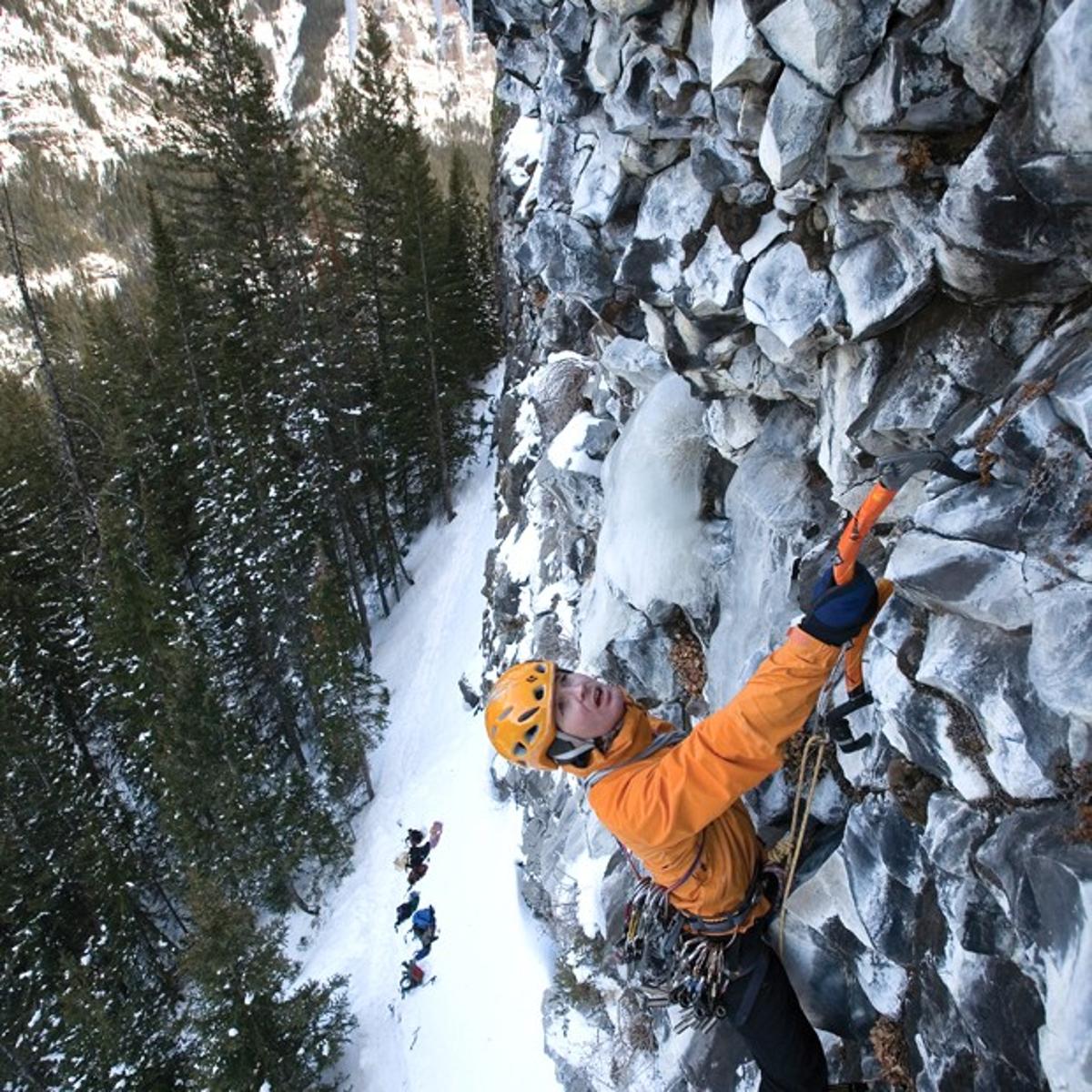In this detailed photograph, a young man in his late 20s to early 30s is captured rock climbing in a challenging winter landscape. He is equipped with a yellow helmet, a yellow jacket, and black pants, and is positioned halfway up a steep, entirely vertical rock wall blanketed with ice and snow. The man is using an orange ice pick, which is lodged into the rock, to aid his ascent and is carefully setting his ropes into the rock for security. His waist belt is adorned with numerous carabiners and other essential climbing gear and ropes. On the left-hand side, a snow- and ice-covered forest of trees provides a picturesque yet harsh background. Below, scattered on the snowy ground between the forest and the rocky mountain, appears to be climbing or camping gear—possibly including an item or person in blue—though it is unclear if others are present or if this individual is climbing solo. Nonetheless, the image vividly captures the intensity and isolation of winter rock climbing.